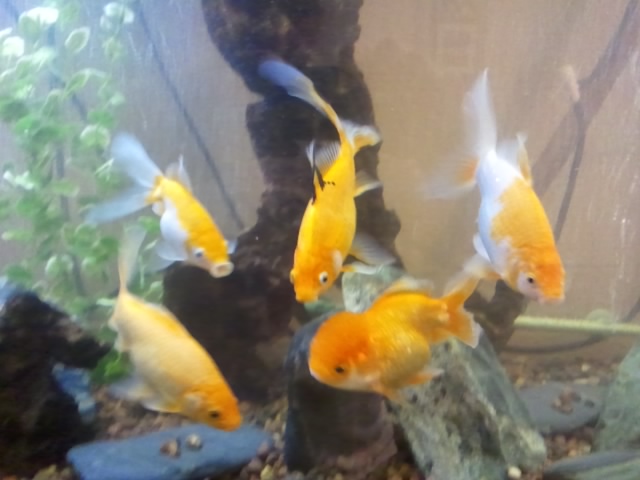The color photograph captures a detailed view of a fish tank. A tall green aquatic plant extends from the bottom to the very top of the tank on the upper left-hand side, while dark-colored gravel covers the bottom. A central rock structure, resembling a small mountain, occupies the middle, surrounded by several smaller rocks. On the far right, a singular air pipe releases bubbles into the tank, and behind the tank, several wires are visible but not submerged.

Within this serene aquatic scene, five goldfish swim gracefully. Two of them are solid gold in color. In the upper left, a goldfish displays a striking white and gold pattern. At the bottom right, another goldfish with a prominent bulbous head can be seen. On the far right, a goldfish with an orange head and mostly white body completes the group. The fish, each about three inches long, mostly swim towards the front glass, bringing vibrant life to the crystal-clear water.